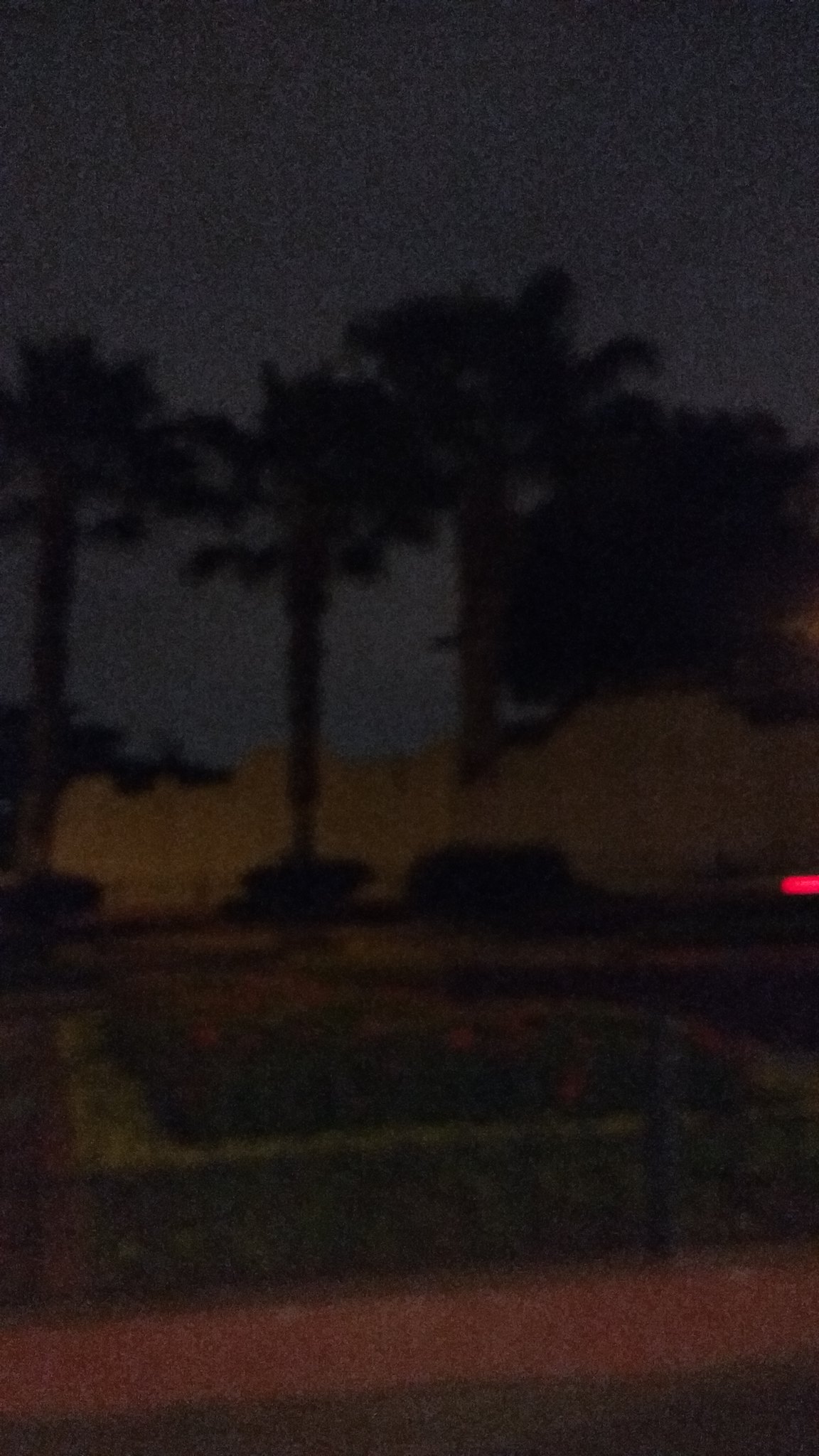In this very dark and dim photograph, the scene reveals a shadowy street or driveway bordered by palm trees and a sturdy white fence or wall in the foreground on the opposite side. The left side of the image shows these towering palm trees with surrounding bushes, their dark silhouettes faintly visible against a near charcoal-black sky that suggests either early sunrise or sunset. In the midsection and right side of the picture, a distinctive red line is noticeable amidst layers of color on the ground that transition from brown to pink to dark brown and light yellowish shades. A short brick retaining wall encloses flowerbeds, adding texture to the landscape. In the background, a large, ambiguous beige structure stands out, possibly a wall or an old building with no lights. The overarching atmosphere is one of stillness and obscurity, heightened by the absence of artificial illumination.